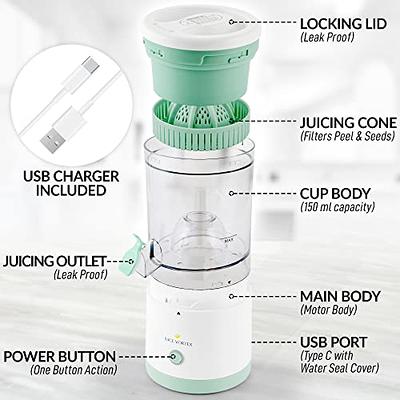This image showcases a detailed, close-up view of a handheld juicer with a clean, predominantly white background to emphasize the product. The juicer is primarily white and teal (or mint green) in color. The device is segmented to display its various parts and features to the customer.

On the left side, there's a close-up inset of a USB charger, with the text "USB Charger Included" below it. Adjacent to this, an arrow points to the left side of the juicer, highlighting a "Juicing Outlet" that is described as "Leak Proof." 

The main body of the juicer, which includes a power button, is white with teal accents. The power button is specified as a "One Button Action" control. The top section of the juicer features a "Locking Lid" that is also leak-proof, ensuring secure operation. 

Inside the clear cylindrical cup body, which is labeled with a 150-milliliter capacity, there's a "Juicing Cone" that effectively filters out peels and seeds. The bottom part of the juicer is the main body, also known as the "Motor Body," where the "USB Port (Type C) with Water Seal Cover" is located.

This comprehensive display accurately portrays each component of the juicer, making it easy for potential customers to understand its functionality and convenience. The juicer is set against a simple white background, accentuating its design and features.